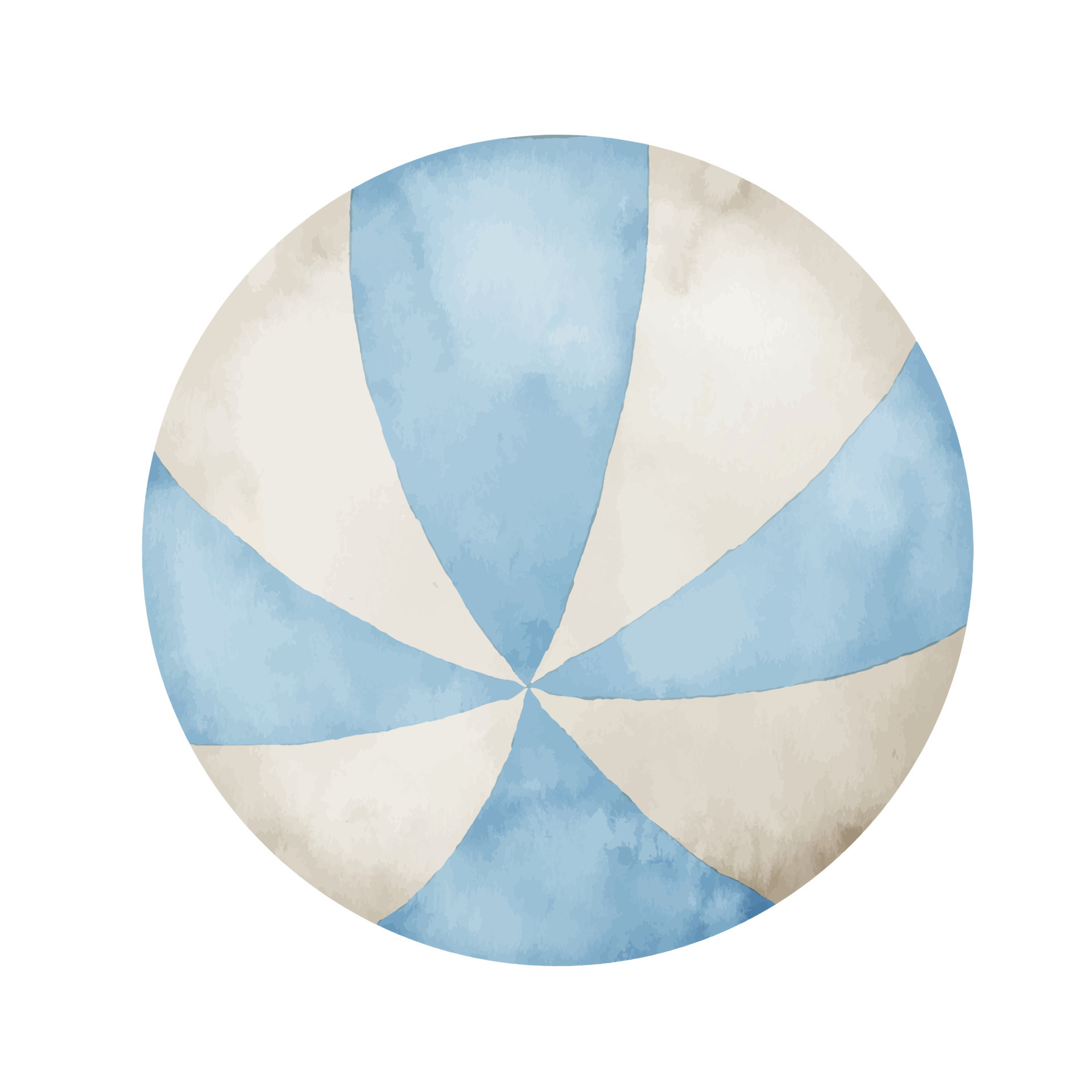This image is a detailed, simple depiction of a spherical ball with no background, set against a plain white backdrop. The ball features an alternating pattern of colors reminiscent of a beach ball or basketball, but with a unique twist in its color palette and design. The ball is divided into eight sections: four light blue and four off-white or grayish-white. These sections are arranged in a pattern where each color alternates, starting from the center and expanding outward, creating a triangular design where the wider ends of the triangles face the exterior of the ball and converge at the central axis on both sides.

The overall design is reminiscent of a hand-drawn or watercolor painting, as indicated by the slightly varied textures and the less-than-perfectly-straight lines that add a soft, artistic touch to the image. The painting lacks any sort of background elements or signatures, focusing solely on the ball itself. The choice of light blue and muted white colors deviates from the usual bright, vibrant hues traditionally seen in beach balls, offering a more subdued aesthetic.